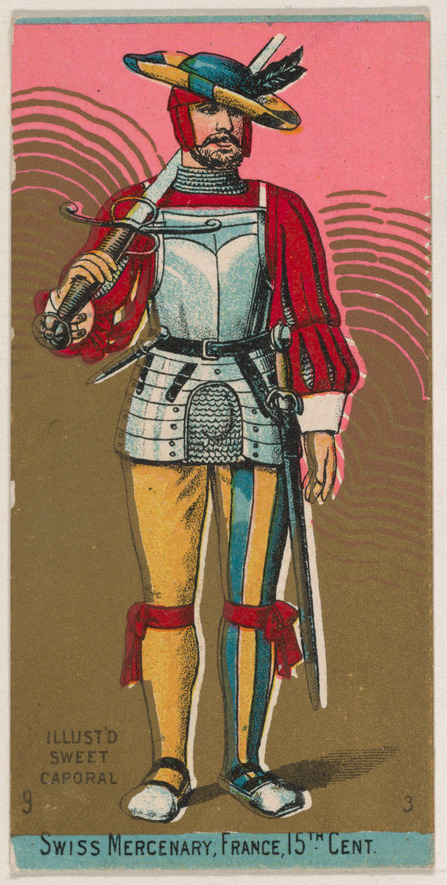This detailed image, possibly a photograph of an old stamp or an illustration, captures a Swiss mercenary from France in the 15th century, as labeled at the bottom of the picture. The caption above reads "Illustrated Suite Kaporal." The mercenary is strikingly attired in a red, puffy Tudor-style shirt overlaid with an apron-like chest plate of steel armor that covers his torso and upper waist. His trousers are vibrant and eccentric: the left pant leg is solely yellow, while the right is vertically striped in green and yellow. Red ties adorn his knees, and he pairs these with silver shoes. Adorning his head is a red helmet topped with a green and yellow striped top hat, from which a black feather protrudes. This headgear sits slightly askew. He holds a large sword draped over his left shoulder and has another blade hanging off his belt at his left side. The background is a mix of brown and pink hues, adding to the historical ambiance of the image.